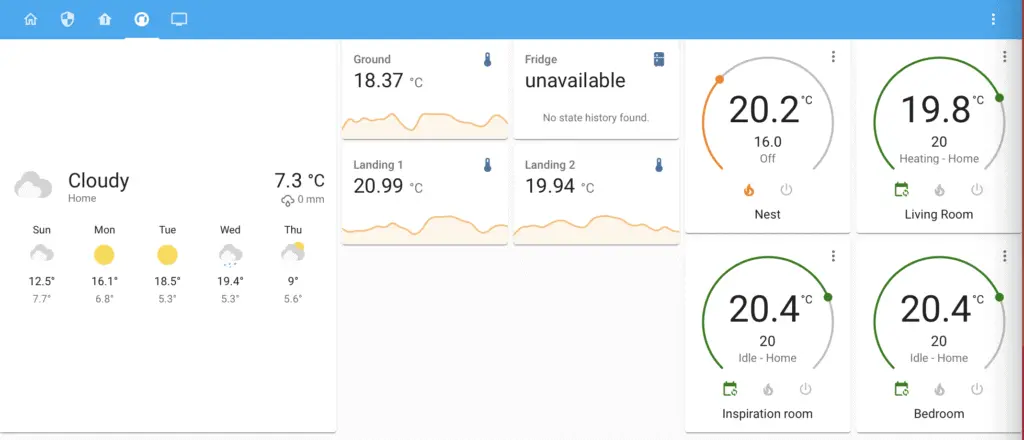The image depicts a weather-based webpage layout. At the top of the page, a blue bar spans horizontally, providing a consistent theme. On the left side, a vertical column of icons includes a home button, an icon resembling a computer, and another circular icon. Additionally, there's another icon similar to the home button. The right side of the blue bar features three vertical dots, likely serving as a menu or options button. 

The main section of the webpage on the left starts with a white box labeled "Cloudy Home" at the top. Below this title, it reports a current temperature of 7.3 degrees Celsius along with a cloud icon indicating cloudy weather. The forecast extends across Sunday, Monday, Tuesday, Wednesday, and Thursday, highlighting that only Monday and Tuesday are expected to be sunny.

Centrally, there are four smaller boxes titled "ground," "fridge," "landing one," and "landing two." Each box, except for the unavailable one, showcases a graph with varying lines and numbered axes ranging up to 10.

On the right side, another set of four boxes is present, labeled "nest," "living room," "inspiration room," and "bedroom." These boxes display temperature readings: 20.2, 19.8, 20.4, and 24.4 degrees Celsius, respectively.